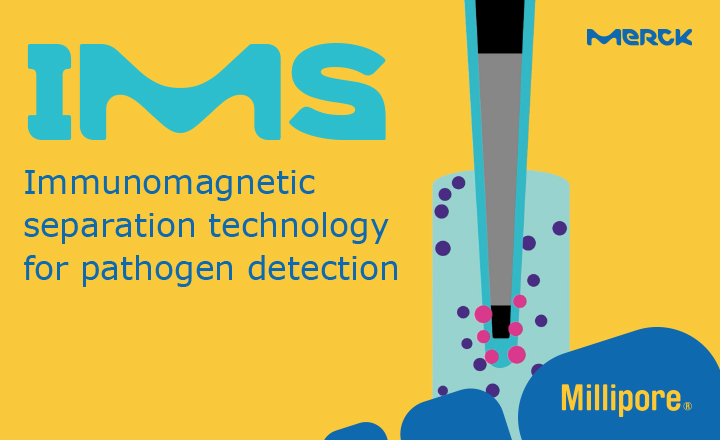The image is a digital advertisement featuring Merck's Immunomagnetic Separation (IMS) Technology for Pathogen Detection. The background is golden yellow, and in the top left corner, large teal letters spell out "IMS." Below that, in modern blue font, it reads, "Immunomagnetic Separation Technology for Pathogen Detection." In the illustration, there is a teal-outlined, long, narrow device resembling a microcentrifuge tube with a micropipette. This device appears to attract and interact with a cluster of dots, most of which are purple, with a few pink ones, representing pathogens. These dots are largely concentrated in the middle and bottom areas of the image. The bottom right corner features the brand name "Millipore" in blue, while the top right corner prominently displays "Merck" in blue text. The overall design suggests advanced pathogen detection technology with the dots being manipulated by the device's separation process.